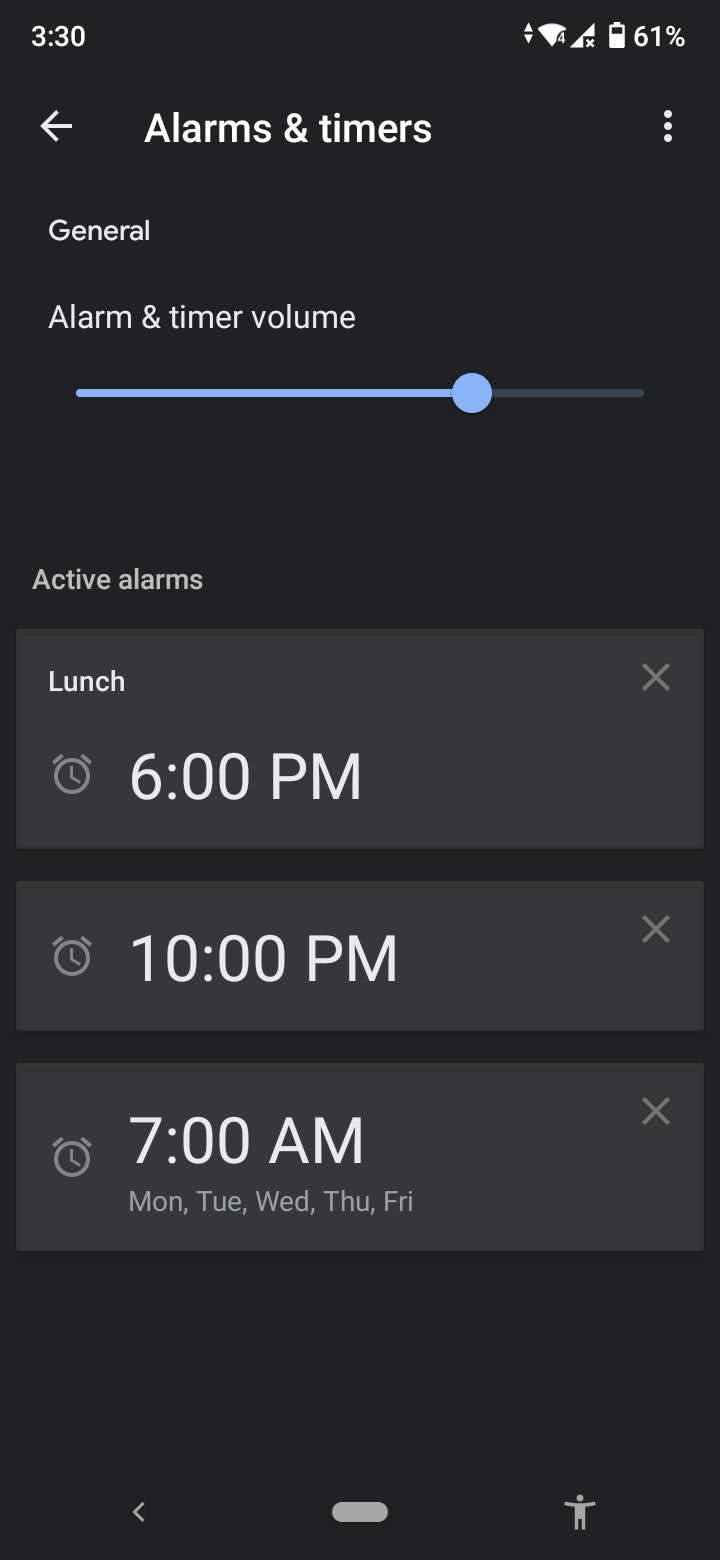The screenshot captured from a cell phone showcases a user interface with a dark background. At the top of the screen, there is white text displaying "3:30" alongside several status icons including a 61% battery indicator, a battery icon, Wi-Fi signal, cellular signal, and an up-and-down arrow symbolizing data transfer.

Below these status indicators, there is a navigation bar. On the left side, a white left-arrow icon is visible next to the text "Alarms and Timers," with "Alarms" capitalized. To the right, three vertically arranged dots representing a menu option are also present.

The screen then displays several sections starting with the text "General" followed by "Alarm and Timer Volume." Below this, there is a blue line with a circular marker indicating the volume level.

In a smaller font, the text "Active alarms" is shown, followed by three alarm panels in dark gray or charcoal. Each panel lists a specific alarm:

1. The first panel reads "Lunch" with an alarm icon underneath it and the time "6:00 PM."
2. The second panel shows an alarm set for "10:00 PM."
3. The third panel indicates an alarm set for "7:00 AM."

For each of these alarms, there is a small "X" icon in the upper right corner, presumably for deleting the respective alarm.